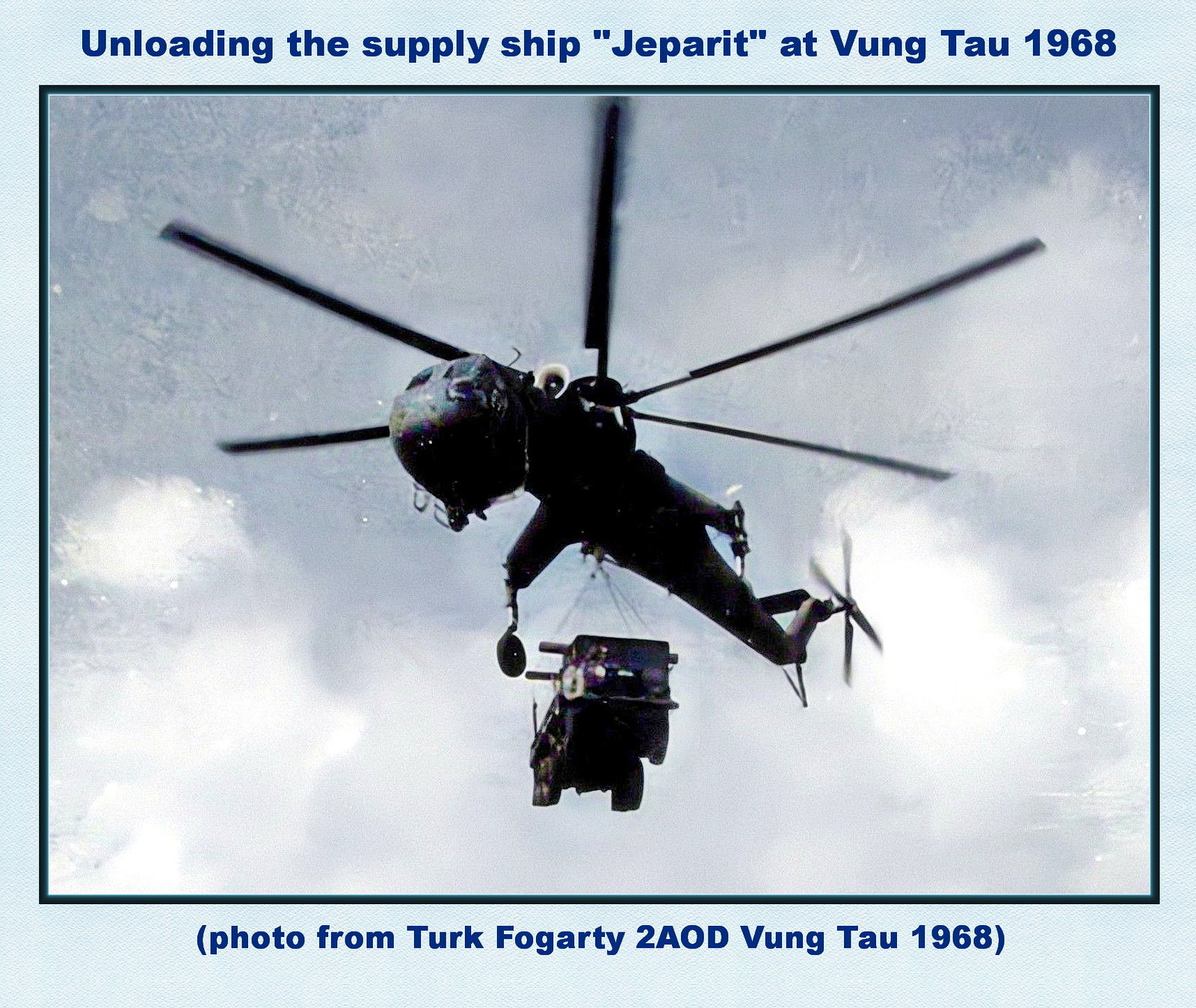This image depicts a historical photograph of a dark-colored military helicopter lifting a smaller vehicle, likely a trained military vehicle, with wires. The scene is viewed from below, capturing the rotor blades against a partly cloudy sky. The photo features a prominent light blue border, with the top text in blue letters reading, "Unloading the supply ship Jeparit at Vung Tau, 1968." The bottom text, also in blue, states, "Photo from Turk Fogarty, 2AOD, Vung Tau, 1968." It creates an impression of an old, meticulously bordered card, with the central photograph framed by a black outline. The overall background hue is light blue, and the entire visual is marked by the colors blue, black, and white. Notably, there are no visible people, additional aircraft, or birds in the photo, emphasizing the isolated action of the helicopter in the Vietnam War era.